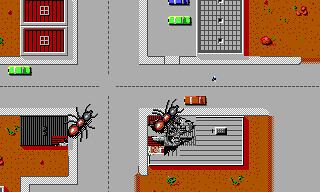In the intricate scene of a video game image, a visually arresting tableau unfolds. At the center-left of the composition, a grayish tree stands prominently, its branches spreading both upward and downward. Meanwhile, in the distant upper right corner, a colorful duo of cars—one green and one blue—can be seen. Positioned around the central part of the image, a series of cross marks add an intriguing focal point. Dominating the right side of the scene is a wide street paved with weathered brown stones, imparting a sense of aged urban texture. An arresting detail captures the eye at the bottom right: a colossal spider or ant-like creature perched atop a building with a gray rooftop, adding an element of suspense and mystery. The area at the very bottom features rich brown wood or flooring interspersed with green patches, set against the street, which itself is demarcated by dashed lines indicative of a traffic lane. The overall composition is both complex and immersive, drawing viewers into a vibrant, dynamic world.